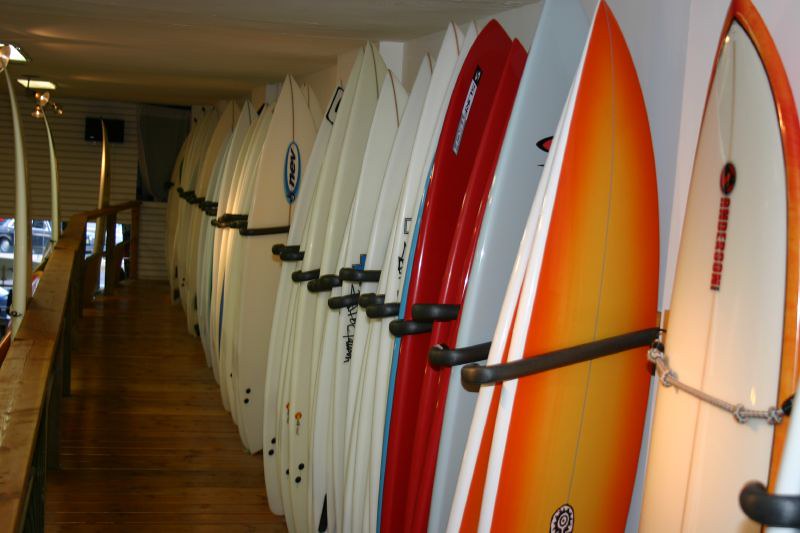This photo was likely taken inside a surf shop, on the second floor. The scene features a wooden platform and railing that acts as a barrier to prevent falls. The space is illuminated by ceiling lights located just a few feet above eye level. Against a white wall, there is a neatly arranged line of surfboards. They are held in place by a black or brown rack system that allows them to be positioned sideways. The surfboards, reflecting light, come in various colors: predominantly white with a mix of orange, yellow, blue, red, and black. Arranged almost in a gradient from white to colorful, one of the notable features is a white surfboard with orange trim facing the opposite direction. There are also some gold-colored poles along the outer side, contributing to the organized yet vibrant aesthetic of the shop.